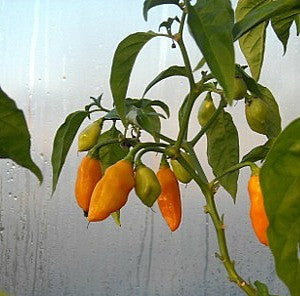The image depicts a thriving pepper plant with a green branch covered in a variety of leaves in different shades of green and light green. Emerging from several branches are peppers at various stages of ripeness, ranging from small, light green and darker green ones to larger, vibrant orange peppers. In total, there are four orange peppers and a similar number of lighter green, still maturing peppers. 

The background features a piece of glass or possibly a plastic lining, characteristic of a greenhouse environment, with visible moisture droplets indicating high humidity. Despite the condensation, the setting appears bright, suggesting it is daytime. Additionally, there is an unaccounted leaf on the far left of the image, potentially from another plant, and a large, hanging leaf towards the bottom right of the frame.